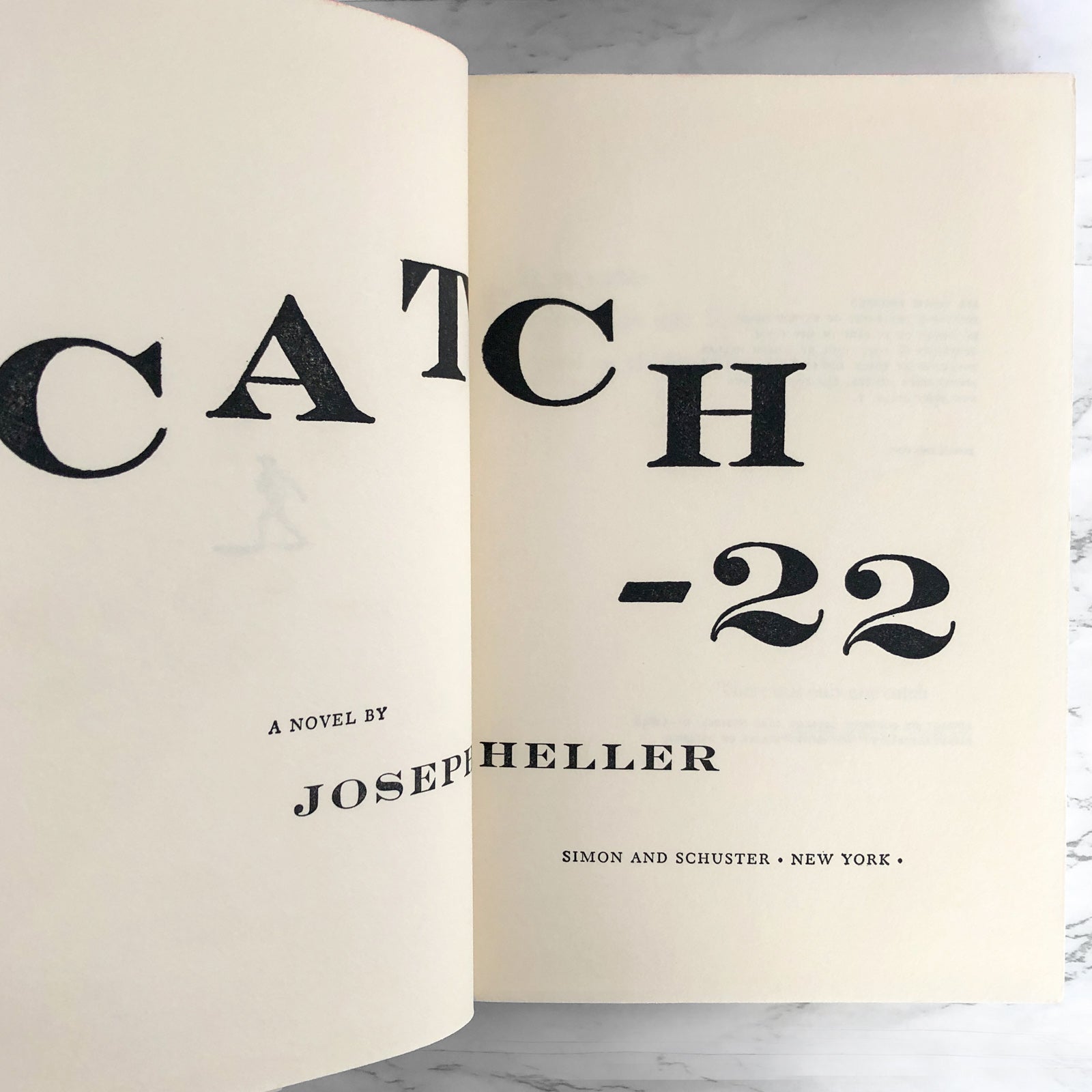This is a detailed photograph of the book "Catch-22" by Joseph Heller, laid open to its title pages on a black and white marble countertop. The book occupies the majority of the frame, with the slightly off-white pages prominently featured. Bold, black uppercase letters span across both pages, forming the title "C-A-T-C-H" on the left page and "-22" beneath the "H." Underneath the title, in smaller text on the left page, it reads, "A Novel By," followed by "Joseph" in larger text. The author’s surname "Heller" continues onto the right page. Near the bottom of the right page, in small print, the text "Simon & Schuster, New York" indicates the publisher. The overall composition emphasizes the book's prominent black text against the minimalist background.